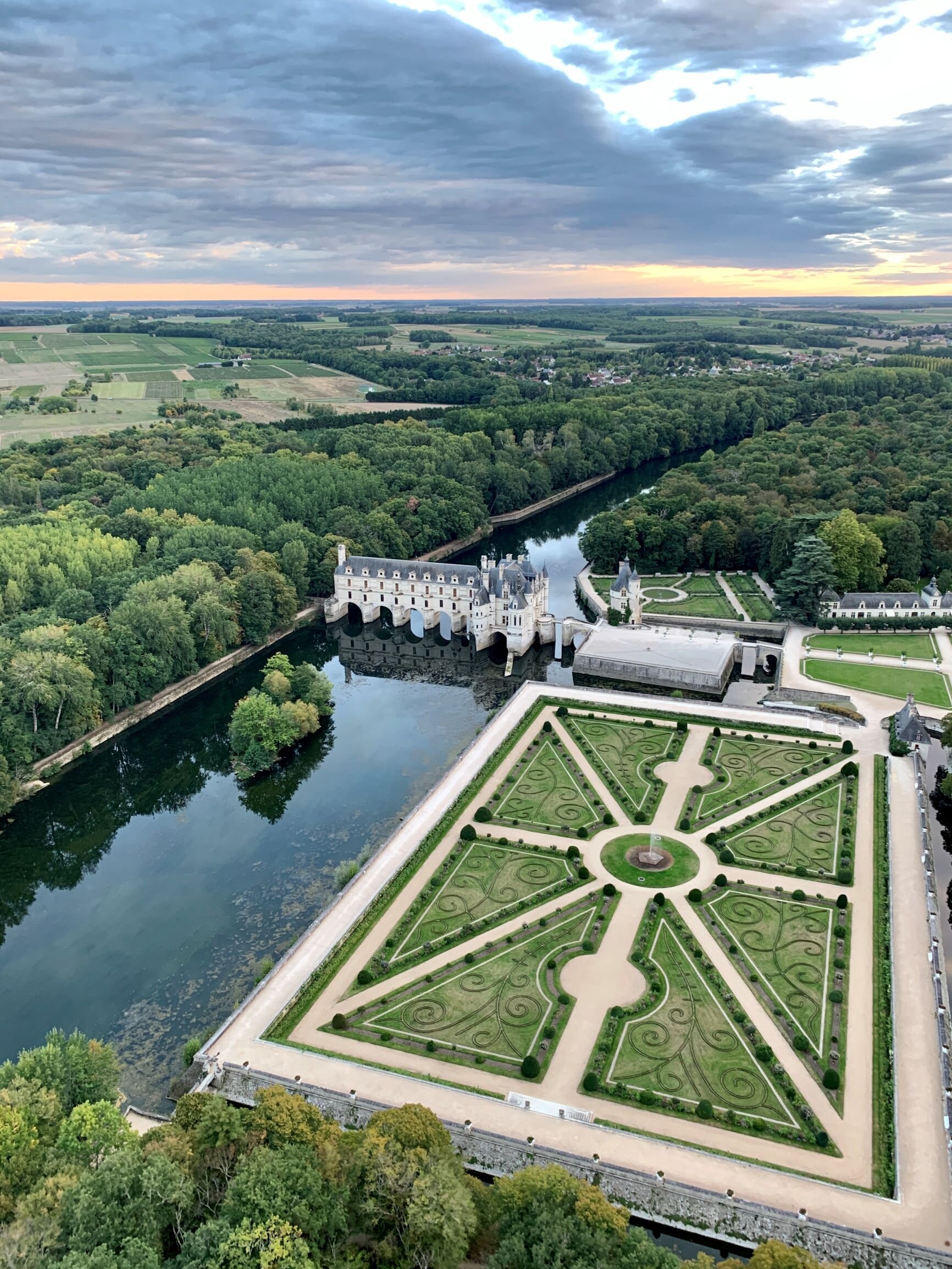This is an aerial photograph capturing the majestic French Château de Chenonceau surrounded by lush greenery and intricate garden designs. The château appears almost as a floating palace, built over a serene stream that flows diagonally across the image from the center left. The château’s foundation is marked by several large archways, designed to allow small boats to pass beneath or dock. This grand structure, with multiple towers and three stories, is a testament to Renaissance architecture.

To the right of the château, there are expansive gardens, meticulously arranged with diamond-shaped sections and curly-Q designs, each converging towards a central circular fountain. This larger, more ornate courtyard is closer to the bottom of the image. Adjacent to this area is a smaller, yet equally impressive building, possibly another part of the estate, characterized by its white exterior and black roof. This secondary structure is surrounded by additional gardens that, while less ornate, contribute to the overall grandeur.

The landscape is richly forested, with thick tree lines bounding the estate on both sides. Farmlands stretch above to the left, leading to a distant city that emerges on the horizon, blending nature's tranquility with human settlement's tranquility and historical significance.